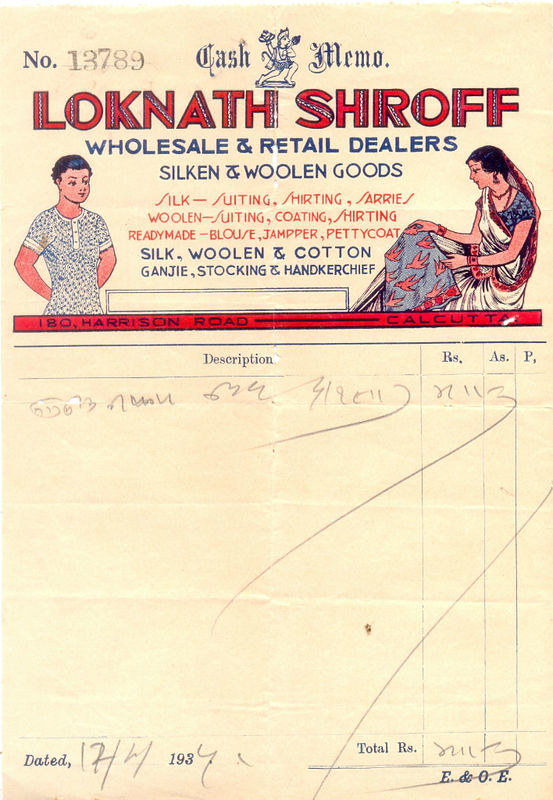The image depicts a vintage-style Cash Memo from India, resembling a magazine page. It features a blend of black and white print with spot colors in red and navy blue. Dominating the top section is a logo reading "Loknath Shroff," identified as "Wholesale and Retail Dealers of Silken and Woolen Goods." The document is titled "Cash Memo" in gothic navy blue print with a small Indian illustration between the words. To the left and right of the logo are images of a man and a woman in traditional Indian attire, the woman notable in a colorful sari and veil, both figures focusing toward the center. The memo bears the crash imprint number 13789 at the top left. Below the logo, there is detailed information about their product offerings, such as silk, suiting, shirting, woolen garments, and ready-made items. The lower two-thirds of the memo contains a layout for item descriptions, prices, totals, and the date, which is hand-marked as 17-4-1987. The overall aesthetic is that of a meticulously crafted piece of vintage print production for business collateral.